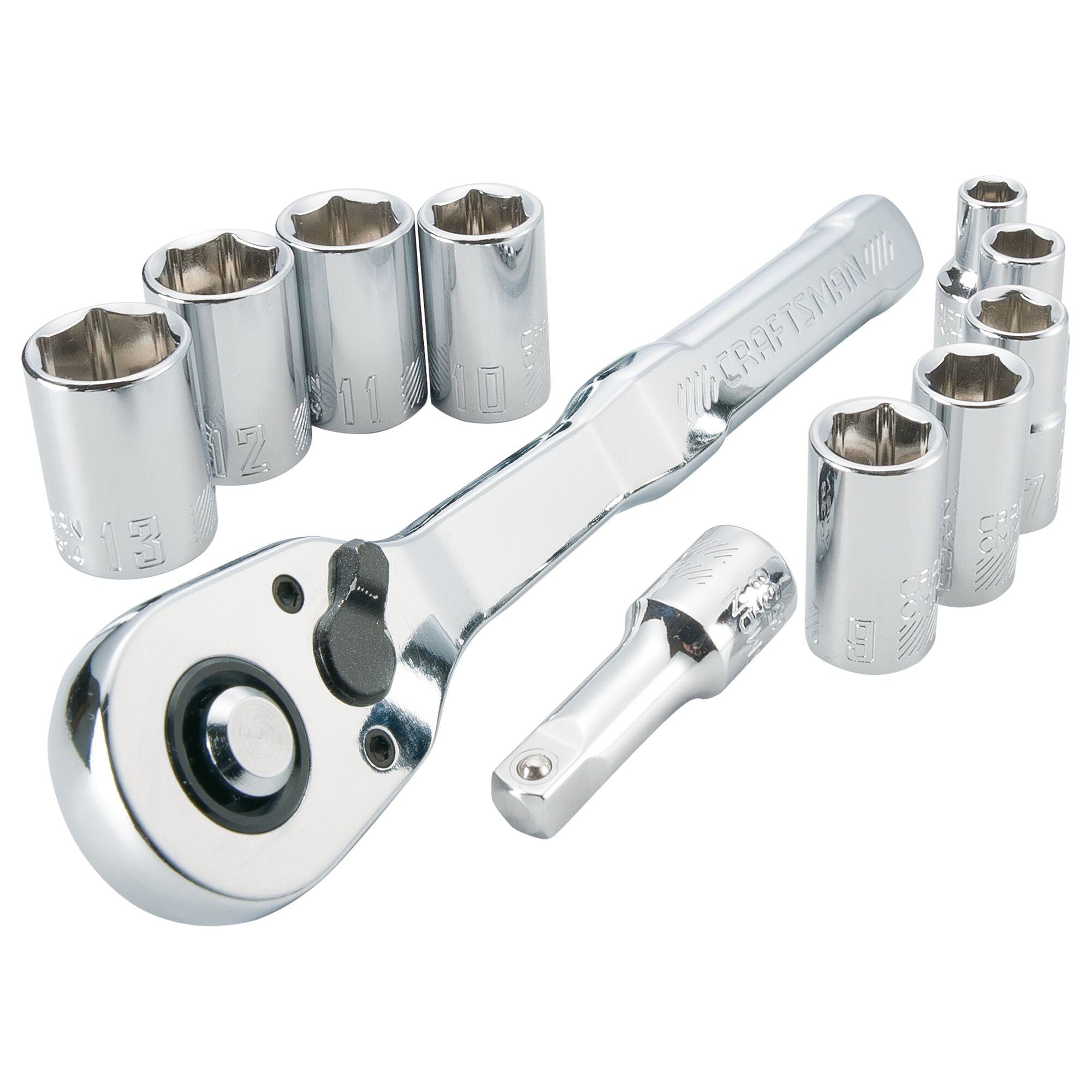The image showcases a professional advertisement for a Craftsman chrome-colored socket wrench set against a pristine white background. Central to the composition is the socket wrench itself, angled slightly downwards with its head facing the bottom right. The wrench is sleek and shiny, with the word "Craftsman" emblazoned on it. It features a small black switch on the ratchet head for adjusting the rotation, and a circular black area with a chrome nodule protruding from it.

Surrounding the socket wrench are a series of socket attachments organized in two neat rows above and below the wrench. These sockets range in size, visibly grading from largest to smallest. The attachments bear size labels such as 13, 11, 10, 8, among others, though some labels are not fully visible. The arrangement emphasizes the precision and variety of the tool set, with the sockets resembling cylindrical shapes akin to larger batteries. Additionally, there is a smaller connector piece that resembles a miniature flashlight or chalice, hinting at its role in extending the tool’s functionality. Overall, the image expertly highlights the new and spotless condition of this comprehensive Craftsman tool set.